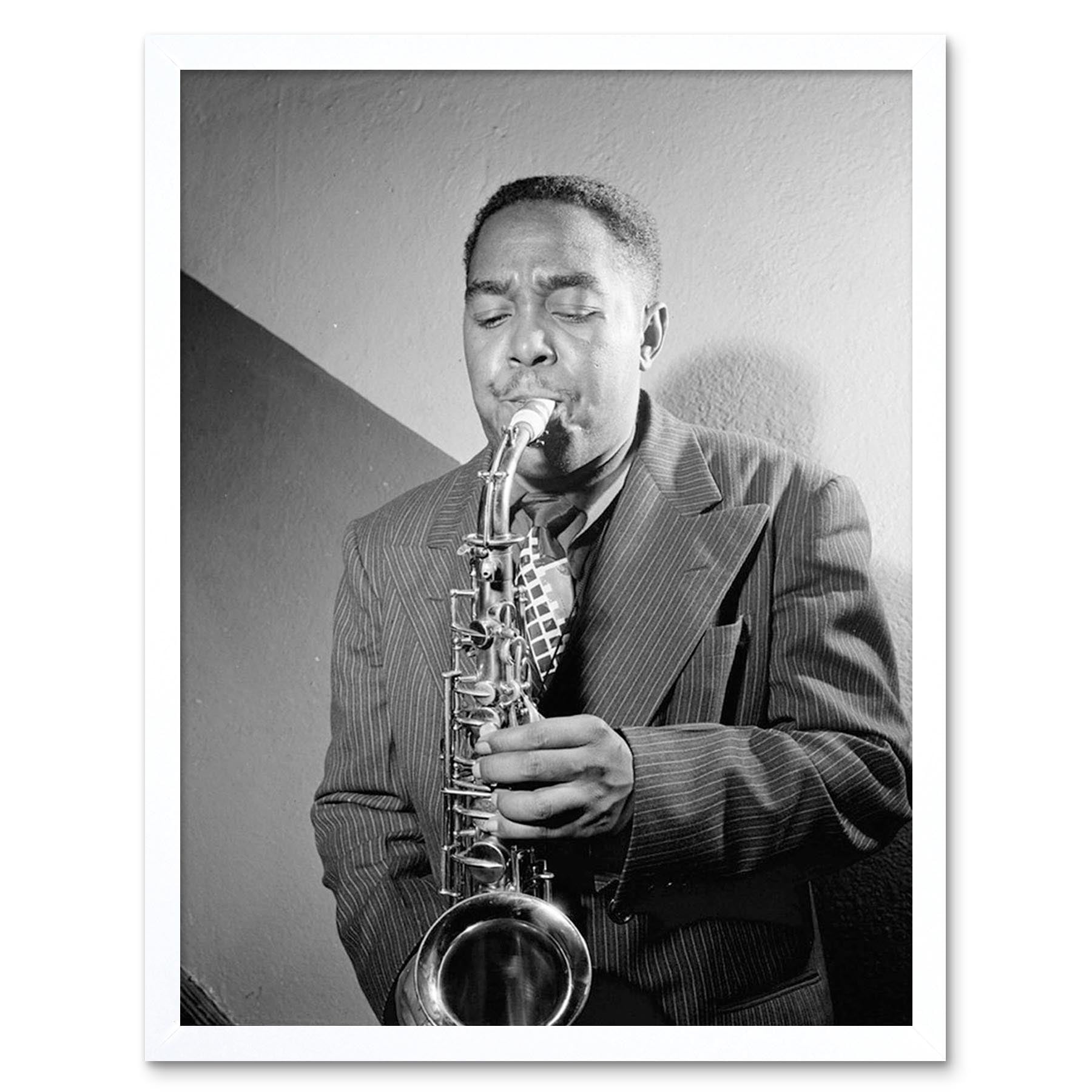A detailed black-and-white photograph in portrait orientation showcases an African or African-American man, approximately in his 40s, deeply engrossed in playing a saxophone. He is dressed in a dark pinstriped suit jacket and a striking, loud tie featuring a white grid pattern, which stands out against his attire. His short black hair and fine, slightly curled mustache frame his face, which appears somewhat chubby, possibly from years of playing the saxophone. The man’s eyes are slightly open, gazing down at the saxophone, projecting a serious and self-assured expression as he loses himself in the music. The image captures him from the waist up, with the open bell of the saxophone visible at the bottom center. The plain background consists of a plaster wall, interrupted by a dark gray diagonal stripe on the bottom left, adding contrast and depth to the otherwise minimalist setting. A subtle light gray shadow cast by the man further enriches the composition.